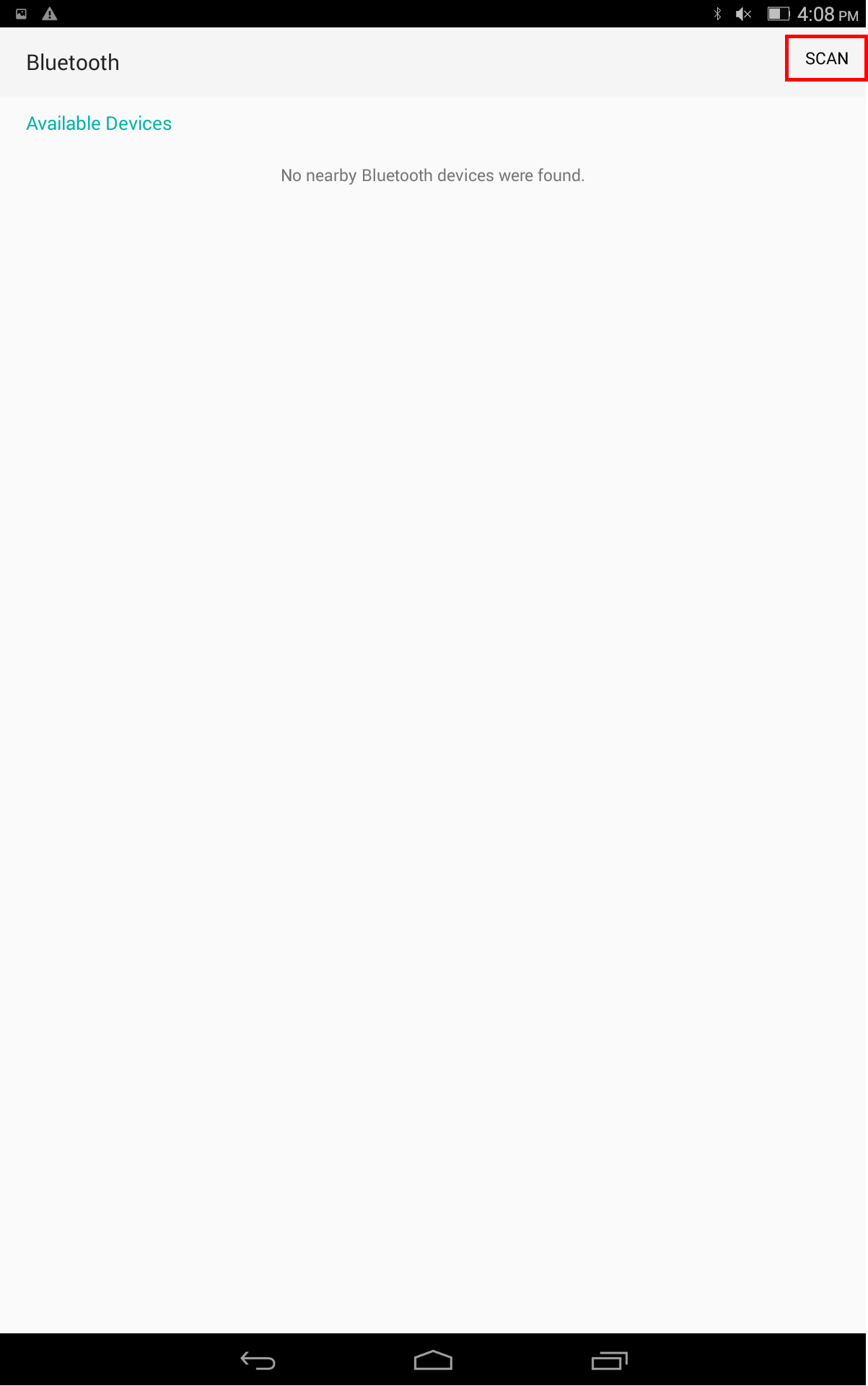The image is a screenshot of an application interface displayed on an Android device. At the very top right corner of the screen, the time is shown as 4:08 PM. Directly beneath the time display, there is a red box highlighting the word "Scan." On the far left of this highlighted section, the word "Bluetooth" is visible. Below this section, the text "Available Devices" is displayed in a neon blue font, indicating a list or section where Bluetooth devices that can be connected to the app are shown. The overall layout suggests that the app is likely used for managing or connecting to Bluetooth-enabled devices.